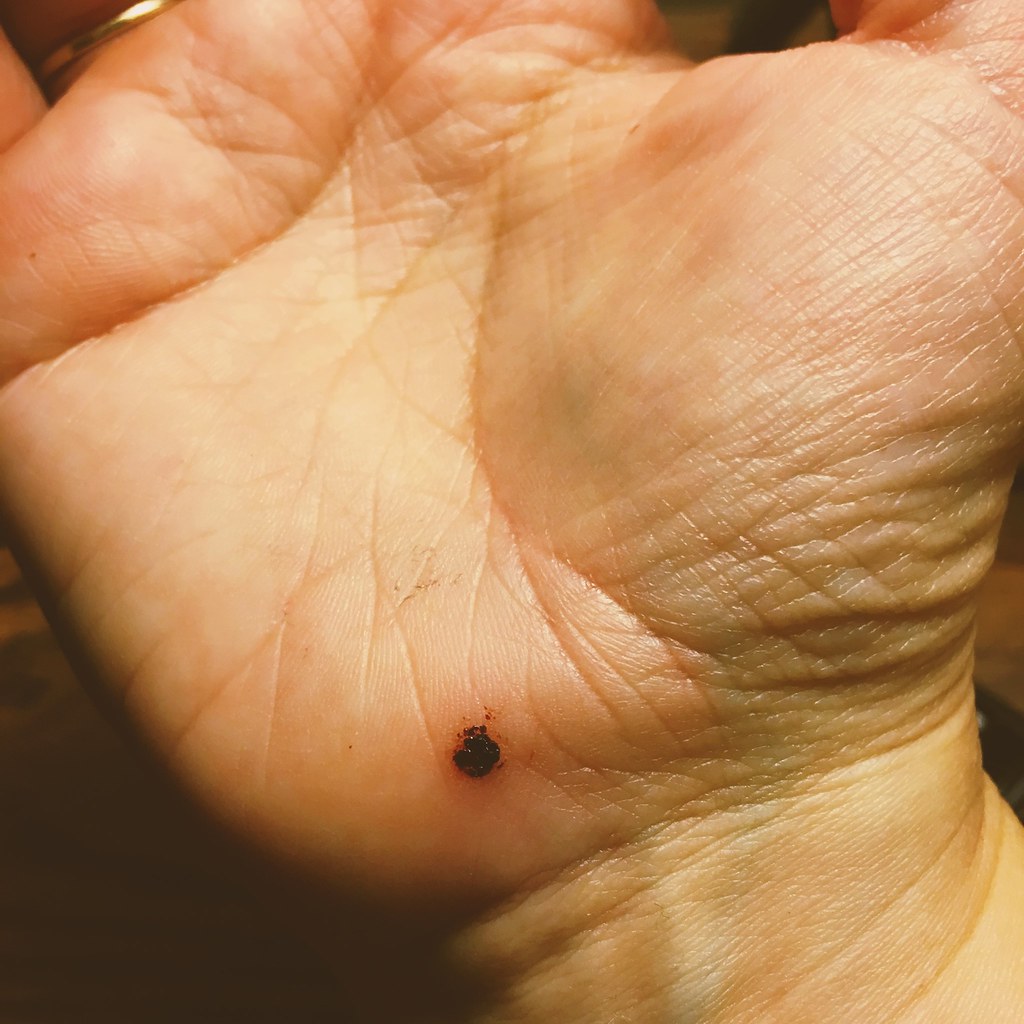This is a detailed close-up photo of a person's right hand, focusing primarily on the bottom of the palm. The hand, which is fair-skinned, is positioned at an angle, with the thumb cropped out on the right side of the image and a partial view of a finger on the left, adorned with a thin gold ring, suggestive of a wedding band. The image captures the intricate lines on the palm and the wrist appears at the lower right corner, while a dark, indistinct background fills the lower left. At the bottom of the palm, near the wrist, there is a noticeable small circular mark. This mark appears black with specks, leaving ambiguity as to whether it is a mole, a healed cut, charred skin, or possibly a burn. The background, though blurred and lacking fine detail, suggests the photo was taken indoors.